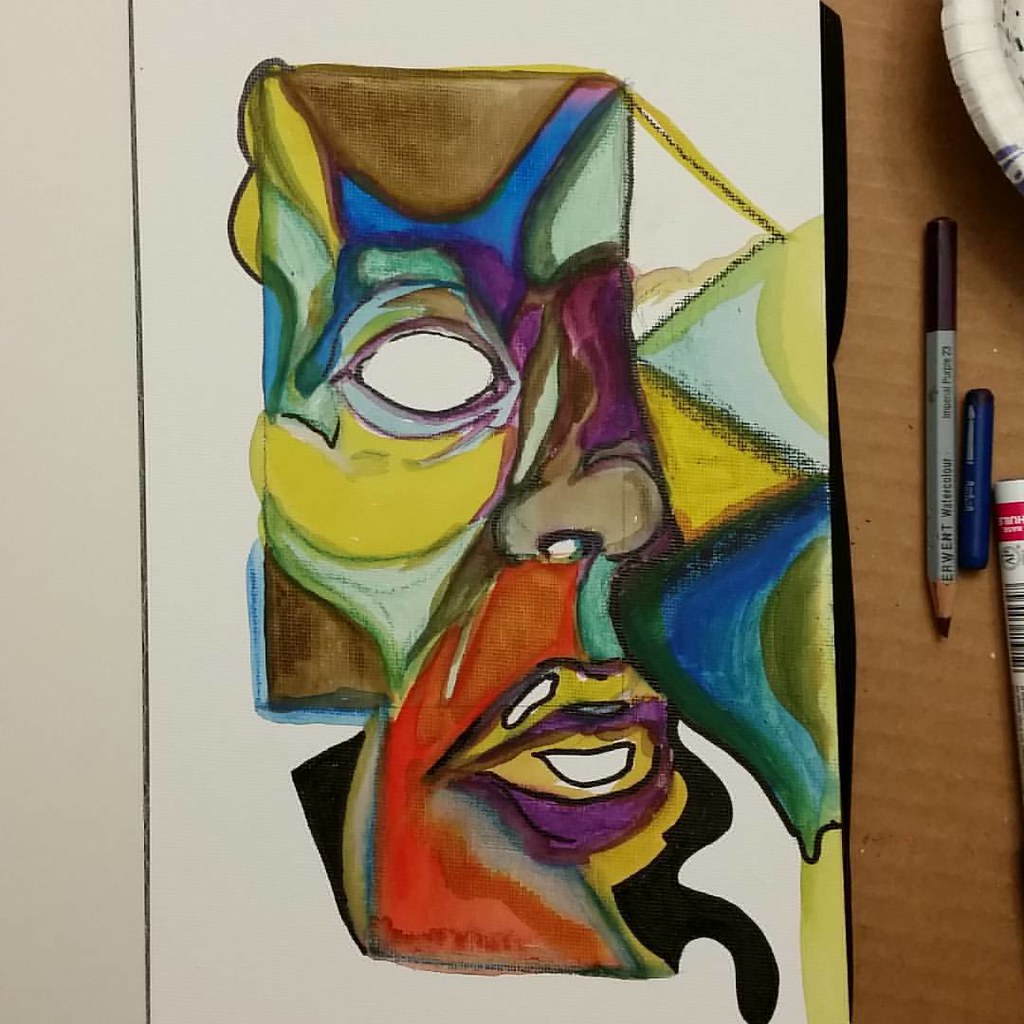The photograph showcases an intricately painted piece of artwork, rendered on what appears to be a white canvas. The vibrant and abstract main image depicts half of a mask-like face, characterized by an eye hole, a prominent nose, and the suggestion of a mouth. A myriad of colors blend together to evoke a festive and whimsical aura, reminiscent of Mardi Gras masks. Surrounding the canvas, on a piece of cardboard, are scattered art supplies including a visible pencil and what seems to be the edge of another pencil or pen. The overall composition juxtaposes the colorful, detailed art with the utilitarian charm of the artist's tools. No text accompanies this visual depiction.